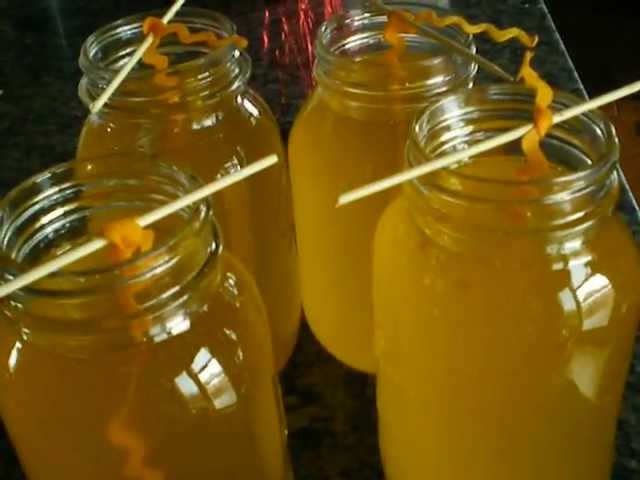The photograph showcases a meticulously arranged setup of four mason jars filled with a yellowish-orange liquid, suggesting some form of a science experiment or homemade infusion. The jars are positioned on a long, black and gray table that extends vertically from the top to the bottom of the frame, bordered slightly by a pitch-black backdrop. Each jar is brimful with the vibrant liquid. A small stick, resembling a toothpick, stretches across the open top of each jar, supporting a piece of orange ribbon or cloth that dips into the liquid, perhaps hinting at the method of infusing the liquid with color or flavor. The setup is symmetrical, with two jars in the front and two in the back, all uniformly designed with the same liquid and decorative stick-ribbon configuration, emphasizing a careful and intentional arrangement.